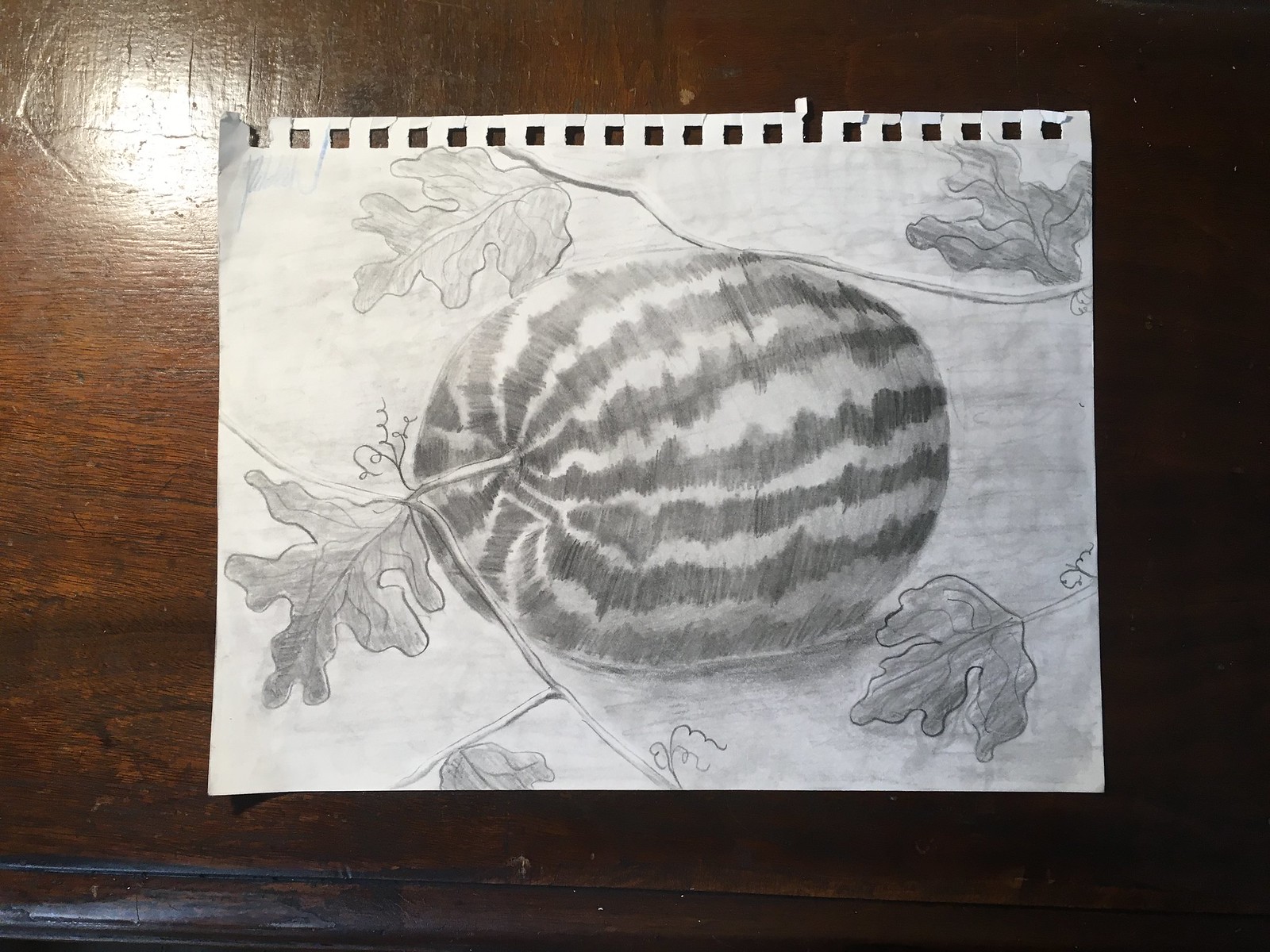This highly detailed pencil drawing captures a meticulously rendered watermelon placed on a piece of paper torn from a spiral-bound notebook. The composition rests atop a reflective, wood-grain table surface. The watermelon, characterized by its horizontally aligned dark and light stripes, lies on its side and is depicted in monochrome shades of gray. A dried, desiccated stem emerges from the top of the watermelon, accompanied by withered leaves. Another elongated stem drapes across the top of the paper, adorned with several more dried leaves attached to stems, adding to the intricate details of the scene. The background is subtly shaded in gray pencil, enhancing the depth and realism of the artwork.